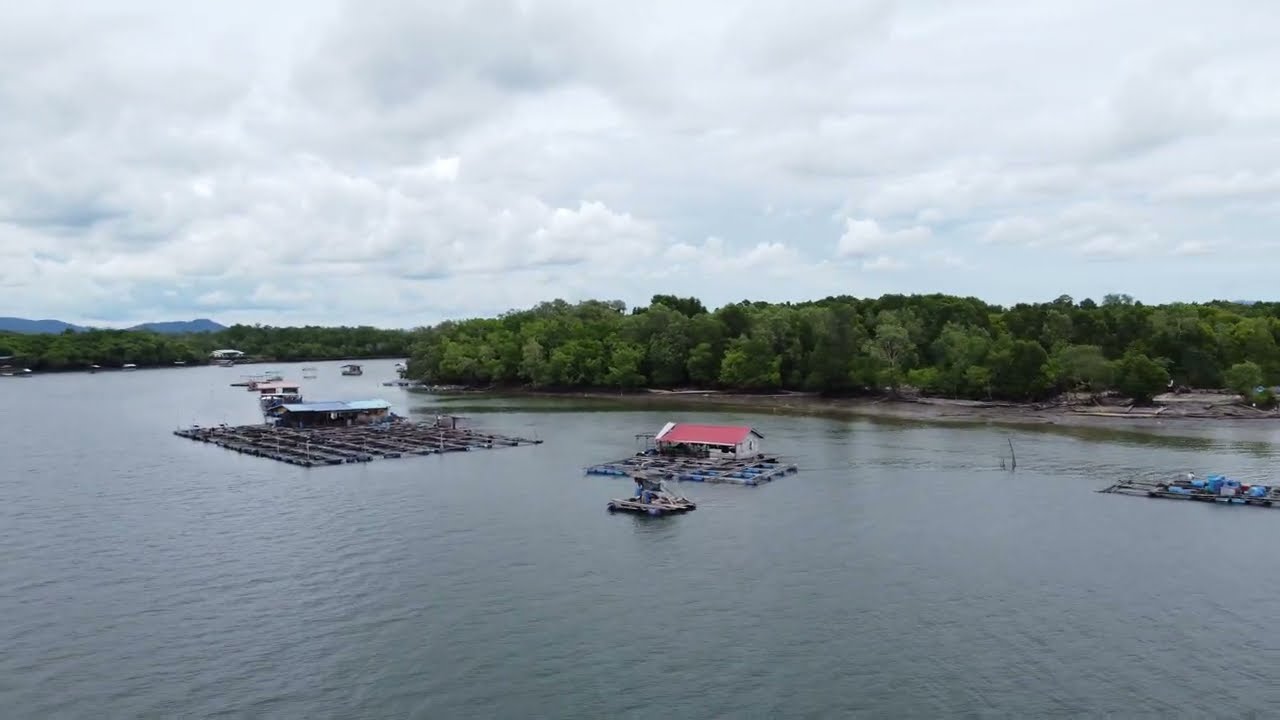In this aerial image, we gaze upon a serene body of water, possibly a bay or lake, characterized by its calm, darkish blue-green hues. At the center of the photo, a series of floating rafts provide an intriguing focal point. These square platforms seem to be constructed atop barrels or pontoons. Each raft supports small structures resembling improvised dwellings; one notable shack features white walls and a distinct red sloping roof, while another nearby sports a green roof. An additional smaller raft is barely discernible and may contain people.

To the left of the image, a large motorboat glides through the waterway, adding a subtle element of motion to the otherwise still scene. The background is dominated by lush green trees blanketing the distant shore, interspersed with glimpses of sandy patches. These trees stretch across the width of the image, eventually blending into a hazy horizon, which may even hint at distant mountains.

The sky above is a tapestry of light blue, heavily adorned with puffy, overcast clouds. These clouds diffuse the sunlight, casting a gentle, subdued light over the entire landscape. The overall atmosphere is tranquil, further accentuated by the absence of visible human activity.